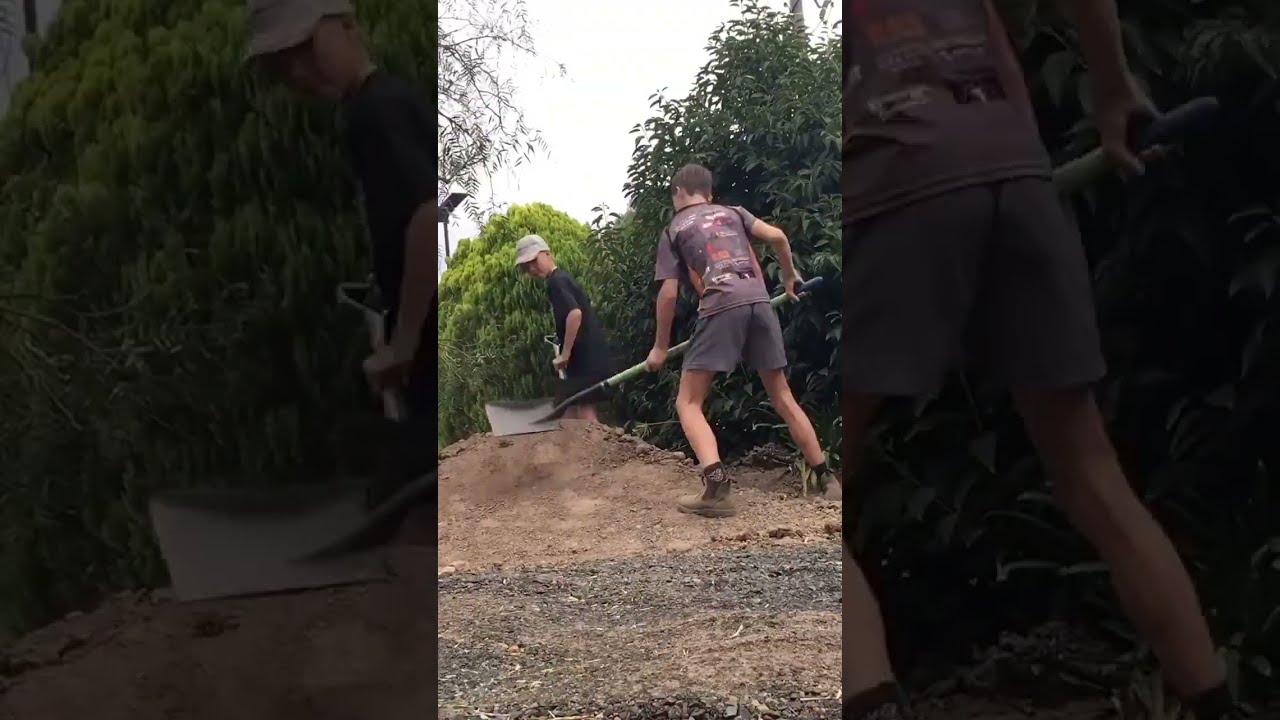This vertical cell phone image, framed by a zoomed-in, faded version of itself, depicts a pair of roughly 10-year-old boys engaged with a pile of lighter brown dirt. The central scene captures the boy on the right standing with his back to the camera; he's holding a square shovel with a green handle on his left side. This boy, characterized by short brown hair and a dark graphic t-shirt featuring cartoons, wears mid-thigh gray shorts and brown work boots. Opposite him across the dirt mound stands another boy, his left side visible to the camera. He's adorned in a black shirt and a tan baseball cap, and he also wields a square shovel, distinguished by a handle with a square grip. The backdrop includes large bushes and small trees, suggesting the boys are possibly working within an orchard or a similarly rustic environment. The ground around the dirt pile is covered in gravel, adding to the outdoor, earthy ambiance of the scene.